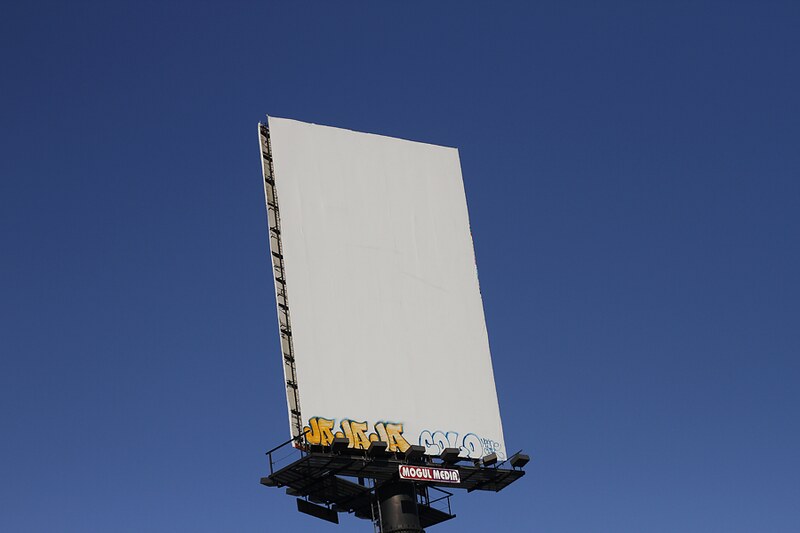Against a clear, deep blue sky devoid of any clouds, there stands a vertical rectangular billboard, predominantly white in color. Near the bottom left corner, there's some graffiti comprising three sets of two bubble-font letters. The insides of these letters are filled with bright yellow. Leftward of this graffiti is an illegible, outlined-in-blue word with white filling. The billboard's structure reveals it to be double-sided, indicated by its narrow V-shaped scaffolding, implying a different advertisement on the reverse side. The billboard bears the insignia 'Mogul Media.'